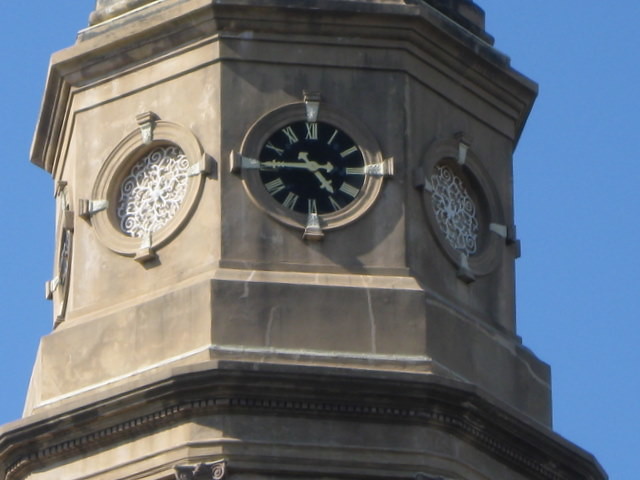This image depicts an outdoor scene featuring an imposing stone clock tower with an octagonal shape. Dominating the frame against a medium blue sky, the clock tower features a large, central clock face with black background and prominently displayed Roman numerals in a tan or gold color. The clock's hands are large and gold-colored, pointing to approximately quarter to five. Each corner of the clock is accented in white, coordinating with the ornamental white swirls and patterns encased in wire mesh that adorn the surrounding circular windows. These swirled circles, unlike the central clock, do not display the time. The overall structure exhibits ornate plinths at the top and bottom, contributing to its grand and historic appearance.